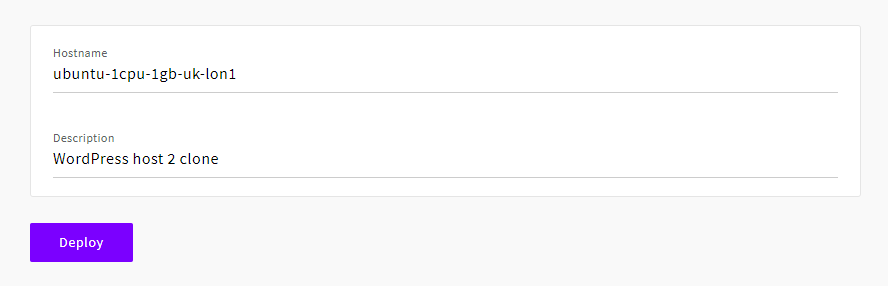The image consists of a horizontally rectangular screen with a predominantly white display area framed by a light blue, almost pale blue, background. The central white rectangular box serves as the main focal point within the image. 

In the upper left corner of this white box, the gray text "Host Name" stands out, capturing attention with its simplicity. Immediately below this label is a sequence of characters displayed in black font: "UBUNTU1CPU1GBUKLON1". This alphanumeric string is both bold and precise, providing key technical details.

Beneath this sequence, a long, pale gray line stretches across the entire width of the white box, acting as a subtle divider. Following this, the word "Description" in gray text designates the next segment. Below it, the phrase "WordPress Host to Clone" appears in black, providing a concise yet informative description of the entity.

Another pale gray line, identical in style to the first, runs horizontally across the white box, creating another visual separation. 

At the bottom of the image, outside the main white box but still within the light blue background, there is a bright blue rectangular button. Inside this button, the word "Deploy" is prominently displayed in white, inviting interaction.